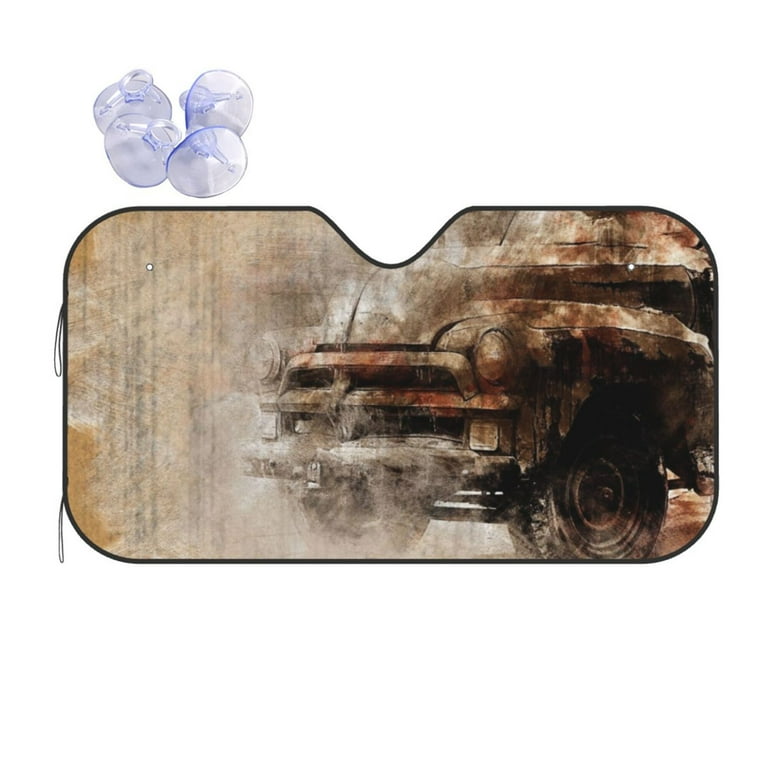The image features a predominantly white background, which serves as a canvas for several distinctive elements. In the upper left corner, there are four small, round, balloon-like figures with gray bodies and bluish tips, resembling tide balloons or suction cups. Below these floating figures, the focal point of the image is a rectangular sign with a top center dip, creating a triangle cutout shape. This sign, outlined in black, displays an artwork dominated by various shades of brown, gray, and beige, evoking a rusty and dirty appearance. The artwork depicts an old, rusted pickup truck facing left with visible details like head lamps, front bumper, and one of the two front tires. The truck seems to blend into the background, which shares the same earthy tones, further enhancing the aged, rustic feel of the image. Two small string pieces can be seen hanging from the left upper and lower parts of the sign. The image's detailed textures and muted color palette create a vintage, weathered look.